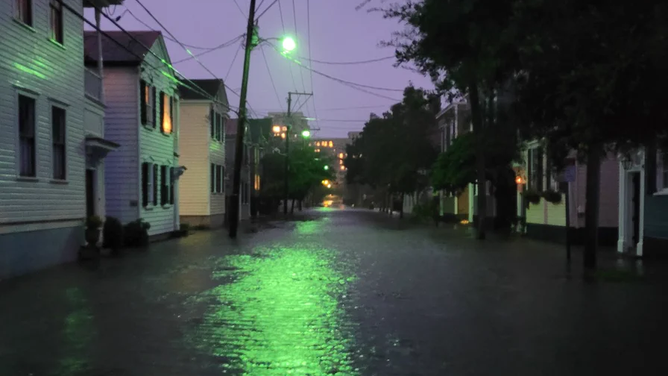This evocative nighttime photograph captures a rain-soaked street lined with rows of small, primarily white houses on either side. The wet pavement glistens with reflections from a green street light, casting various shades of green on the ground. Telephone poles and crisscrossing wires span the top part of the image, adding to the serene yet intricate scene. Several houses have their windows and porch lights on, casting a warm glow against the moody backdrop. The sky, a mesmerizing lavender hue blending into blue, features a clear, circular moon. In the background, a ten-story building with some illuminated windows rises above the line of houses and trees, which flank the street. This tranquil scene is devoid of people, allowing the viewer to fully absorb the peaceful, rainy night.